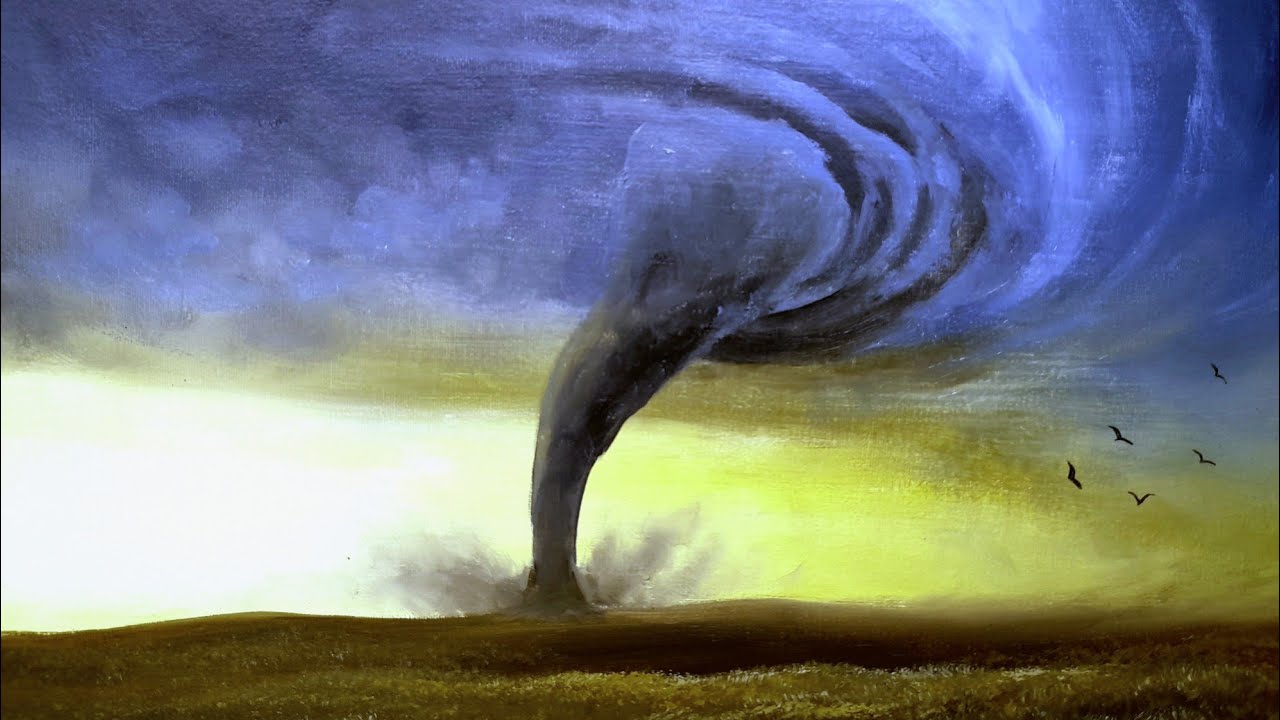This detailed oil painting depicts a menacing tornado tearing through a landscape. The top two-thirds of the canvas are dominated by dark blue and black hues, blending into a swirling mass that forms the upper part of the tornado's funnel. The tornado's core is painted in ominous shades of black and gray, showcasing its destructive power as it touches down, ripping up everything in its path. In the center, the funnel continues downward in dark gray tones, with gray dust and debris being violently ejected from its base.

The painting's backdrop features an eerie mix of ochre, light yellow, and pea-green colors, likely representing dirt and debris caught up in the storm. In the foreground, the ground displays a dark brownish-yellow hue, evoking a flat, barren field. This area includes small patches of grassy terrain interspersed with what appear to be delicate white flowers, suggesting a brief respite from the devastation above.

Adding to the sense of urgency and chaos, several black silhouettes of birds can be seen frantically flying away from the tornado, concentrated mostly on the right side of the image. Their stark, dark forms contrast sharply with the tumultuous, colorful sky, underlining the dramatic escape from the impending disaster. The overall scene is one of dynamic energy and impending doom, capturing the viewer's attention with its vivid portrayal of nature's raw power.